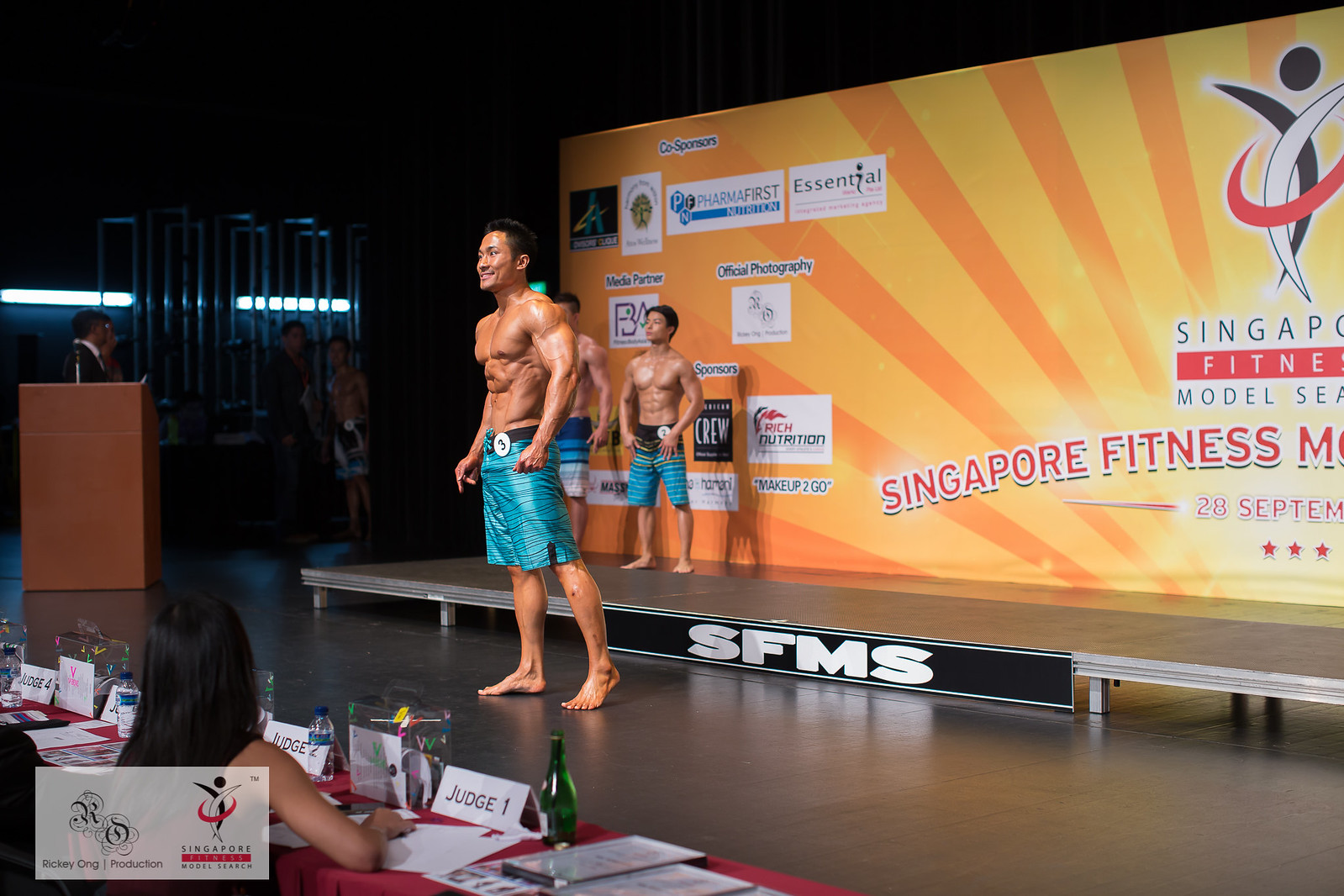The image captures a vibrant fitness competition set against the backdrop of a stunning sunset or sunrise alternating between orange and yellow hues. Dominating the backdrop, the words "Singapore Fitness Model Series" are displayed prominently, although the lower part of the text is cut off at the edges of the frame, revealing only "Singapore Fitness M," and the date "28 September." Above this text is a biomorphic emblem symbolizing the event. At the bottom of the stage, the SFMS logo is clearly visible.

In the foreground, a muscular man of Singaporean Asian descent, wearing blue swim shorts and a number 3 logo on his waistband, stands off the stage. Behind him, two more well-developed men of Eastern Asian descent stand on the stage, wearing similar blue shorts with the man on the far left bearing a number 2 on his belt.

On the bottom left-hand corner of the image, a judge's table is partially visible. The table hosts a female judge with long, black hair, identified by a placard as Judge 1. Additional placards for Judge 2, Judge 3, and Judge 4 can also be seen, although the judges themselves are not visible. The corner of the image also shows a small box with the inscription "Ricky Ong Productions," and it appears to read "Singapore Model Search," hinting at the organizers of the event. Overall, the scene is clearly set in an interior space, structured around the competitive display of bodybuilding and fitness.